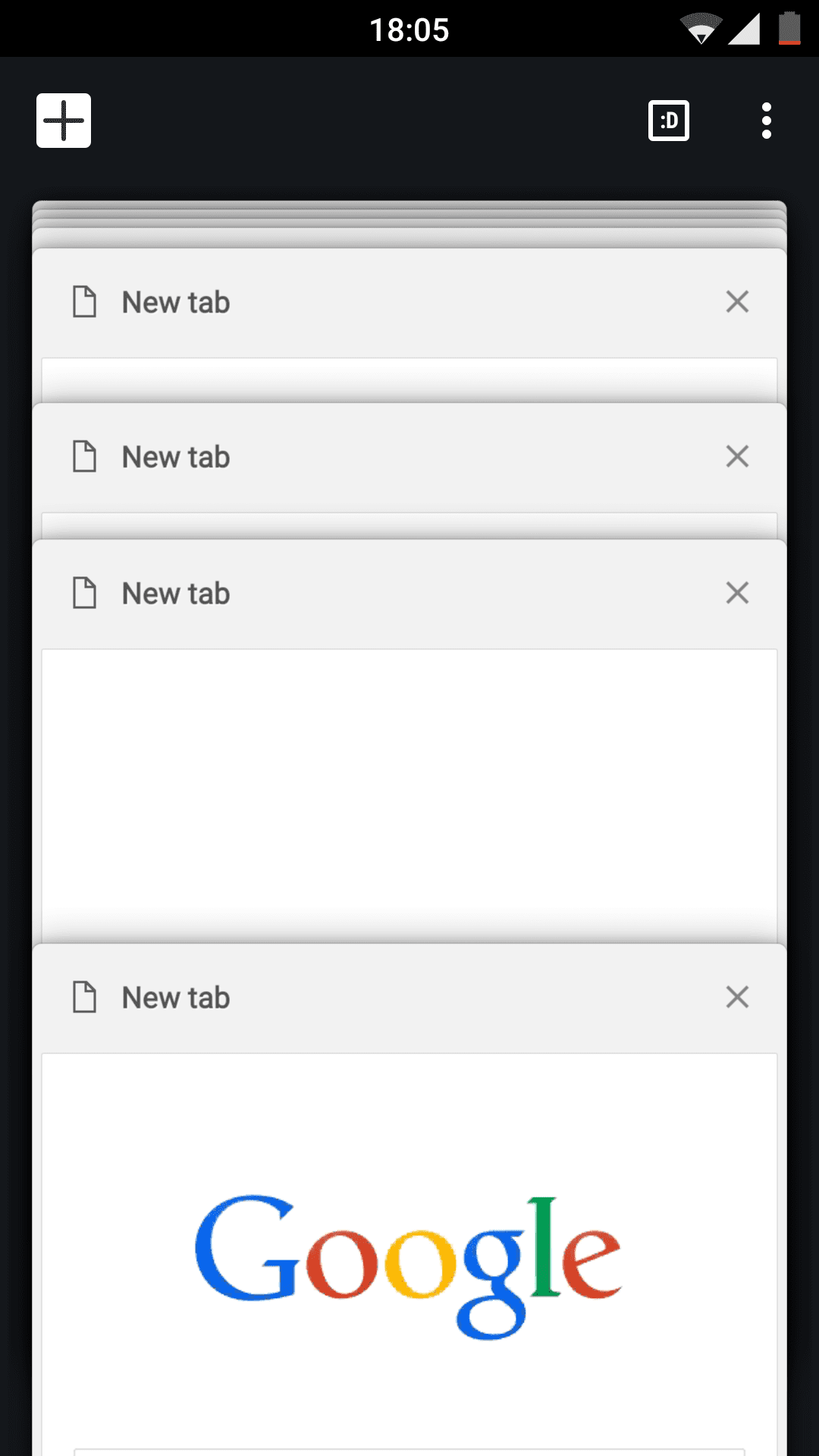The image showcases a smartphone screen displaying a browser interface. At the top of the screen, the status bar indicates the time as 18:05 alongside icons for Wi-Fi signal strength and battery life on a black background. Below the status bar is a toolbar featuring a black "plus" sign on a white background for opening new tabs, a square-shaped button, and a circular button with a colon followed by the letter "D" (possibly an emoji or shortcut). There is also a button with three vertical white dots, likely for additional options.

The primary portion of the screen is dominated by multiple browser tabs. Four visible tabs are labeled "New Tab," each with a piece of paper icon and a grey "X" for closing the tabs. The bottom-most tab shows the Google logo in blue, red, yellow, and green colors on a white background, indicating the Google search page. There are additional tabs visible in the background. The interface has black borders along the edges, while the content within the tabs features a predominantly white background.